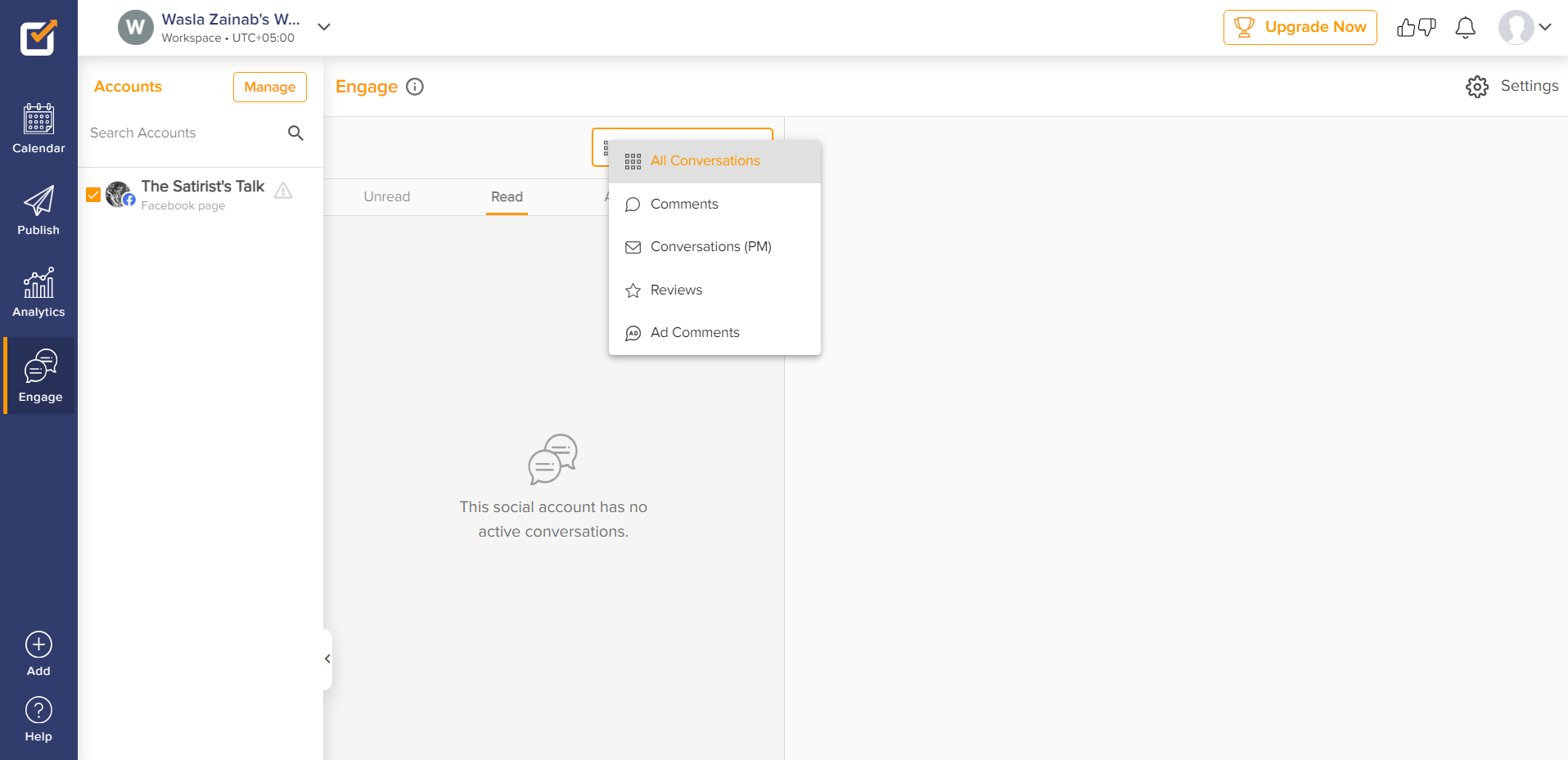This image is a screenshot of Wasla Zainab's workspace interface. On the left side, there's a vertical blue navigation bar featuring several options. At the top is a box with an orange checkmark and an arrow. Below this is a menu with the following options: Calendar, Publish, Analytics, and Engage, which is indicated with two chat bubble icons. At the very bottom are the Add and Help options.

In the top white space, the title "Wasla Zainab's W..." is displayed. Below this, it reads "Workspace UTC+5," accompanied by a gray circle with the letter "W" and a down arrow to the right. On the far right, there is an orange "Upgrade Now" button in a rectangle, along with a plus icon, a feedback icon, a notifications icon, and a profile/account icon featuring a gray and white head silhouette with a down arrow.

Beneath Wasla Zainab's name is a wide white rectangle labeled "Accounts" and "Manage" in orange, both encased in an orange box. Below this, the text "Search Accounts" appears with a magnifying glass icon to the right. Further down is a section divided by a line, showcasing "The Satirists" and "Satirists Talk" on a Facebook page. This section features a gray information icon, an orange checkmark in a tiny square, and a profile image with an "F" denoting Facebook.

To the right of the Engage section is a wide gray box nearly as tall as the white rectangle next to it. It is titled "All Kinds of Conversations" within an orange box at the top and includes categories such as Comments, Conversations, PM, Reviews, and Ad Comments. However, there is no active content in this box. Additionally, the main rectangular area on the right side of the workspace is entirely empty, indicating no active conversations or data displayed.